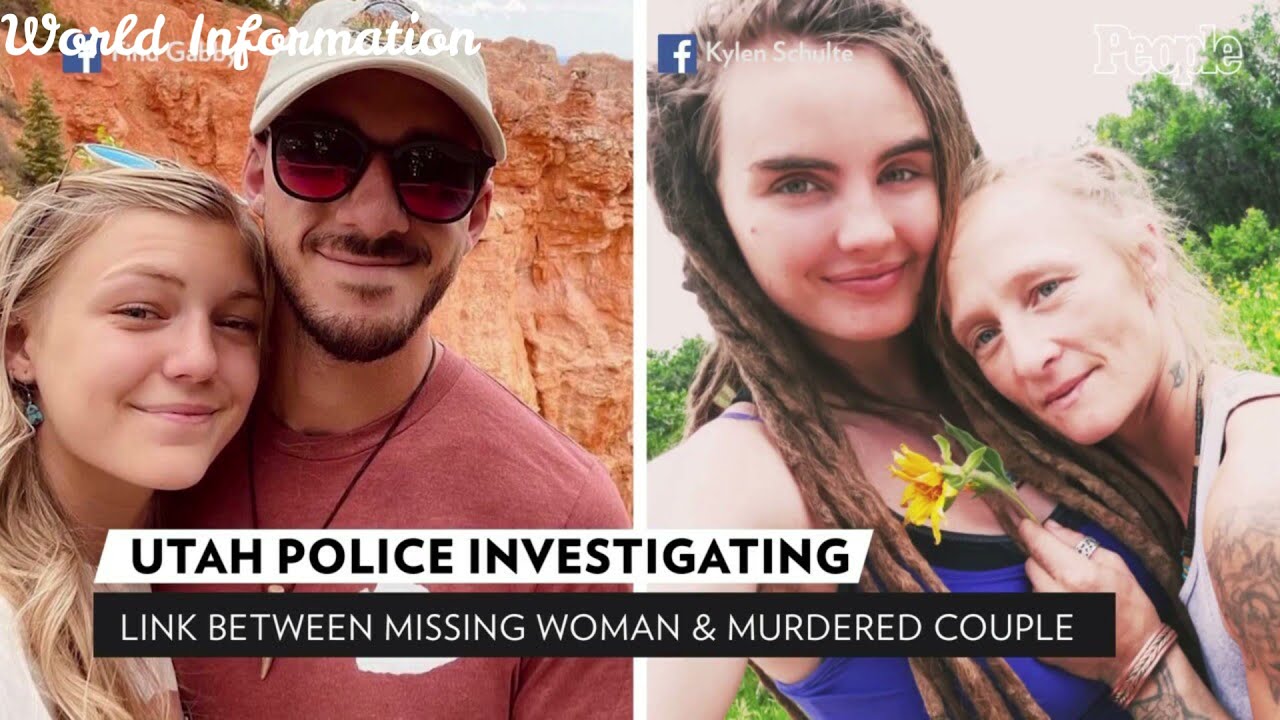This is a detailed screenshot of a news article from what appears to be the website of People magazine, given the "People" logo in the upper right corner. The article is under the "World Information" section, as indicated by a fun, bubbly white cursive font on a rocky, mountainous background with a tan hue and a green tree.

The headline, displayed at the bottom, reads "Utah police investigating link between missing woman and murdered couple" in bold black letters on a white background with a secondary subline in white letters on a stark black background.

The image contains two photos side by side. On the left is a picture of Gabby Petito and her boyfriend, Brian Laundrie, standing in front of red cliffs or a rocky structure possibly reminiscent of the Grand Canyon. Gabby Petito, the blonde woman, is wearing blue-framed sunglasses on her head and earrings, while Brian Laundrie, a man with a goatee, is sporting a white hat, black-framed pink sunglasses, a black necklace, and a maroon shirt.

The right photo features two women. The left woman has light skin, dark brown dreadlocks, and is wearing a blue tank top. She is identified as Kylan Schult from the text overlay. Next to her is an older woman with blonde hair, noticeable tattoos on her arms and shoulders, holding a yellow flower with a green stem, and wearing a white tank top. The pair appear to be close and affectionate in this outdoor setting.

Alongside these images are Facebook logos and names, with one clearly reading "Kylan Schult" and another possibly saying "Find Gabby," indicating a connection to social media and highlighting the ongoing public interest and search efforts related to these individuals. The overarching theme centers on the investigation by Utah police into the potential connection between a missing woman and a murdered couple.